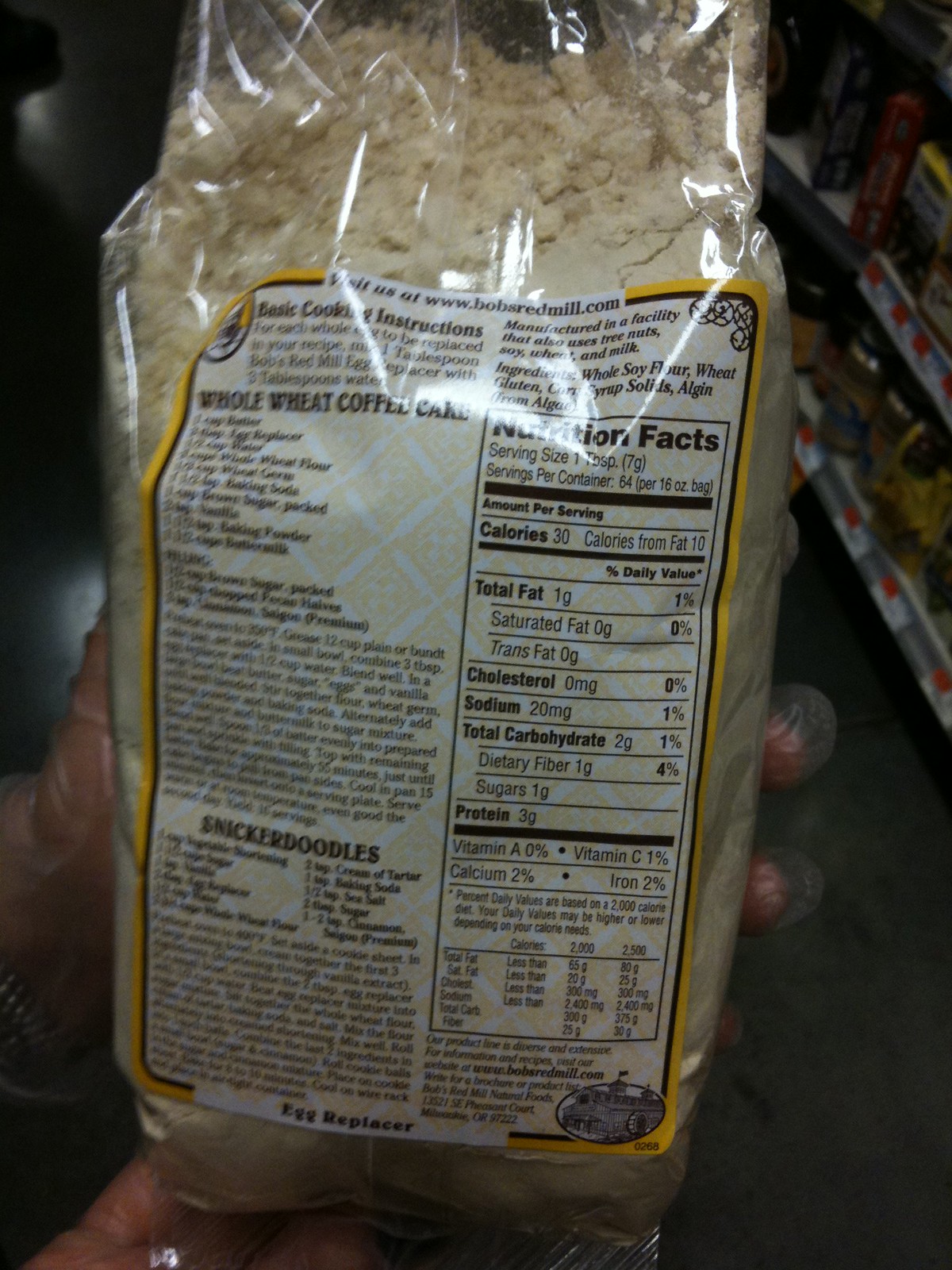In this image, a Caucasian individual is holding a large bag of cookie mix in their gloved hands, providing a hygienic display of the product. The transparent gloves ensure the integrity of the bag's contents is maintained. The bag, predominantly filled with a beige powder, is held against a backdrop of a grayish floor, along with some shelves visible in the top right corner, stocked with various jars and food items, indicating a grocery store setting.

The bag's nutritional label, bordered in yellow, is clearly visible. On the right side of the label, nutritional facts are meticulously listed. To the left, there are two detailed recipes: one for whole wheat coffee cake and another for Snickerdoodles. The top right section of the label features the list of ingredients, while the top left portion provides basic cookie instructions, offering a comprehensive guide for prospective bakers.